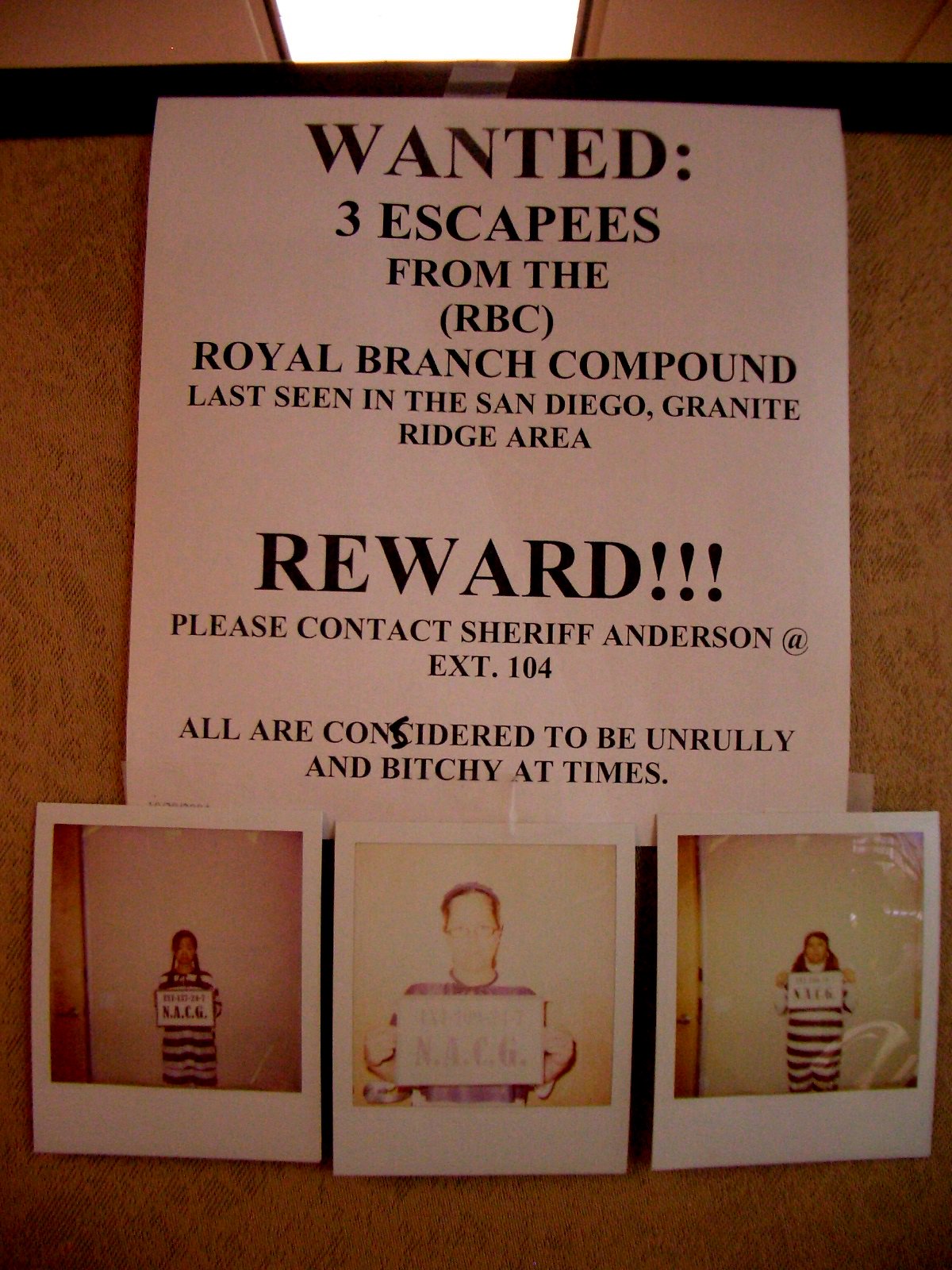This image depicts a satirical wanted poster hanging on a bulletin board. The poster, printed on white paper with solid black, uppercase text, reads: "WANTED: 3 ESCAPEES FROM THE RBC ROYAL BRANCH COMPOUND. Last seen in the San Diego Granite Ridge area. REWARD!!! PLEASE CONTACT SHERIFF ANDERSON AT EXTENSION 104." The notice humorously describes the escapees as "unruly and bitchy at times," although "unruly" was originally misspelled with two L's and "considered" was corrected from "concidered." 

Beneath the text, there are three Polaroid photos of women dressed in black and white horizontal striped outfits, resembling prison uniforms. Each woman is holding a sign with text that isn't fully legible but includes sequences like "N-A-C-G" and a number. The faces in the photos are not clearly visible, contributing to the poster's playful nature. The pictures appear to be taped to the bottom of the poster, adding to the casual, tongue-in-cheek presentation of the "wanted" notice. The background is suggested to be cardboard, and the overall feel of the image suggests it could be an office joke.